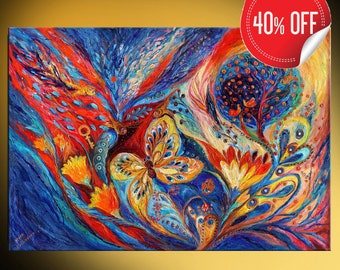The image portrays a vibrant, slightly abstract oil painting featuring a butterfly amidst flowers and perhaps a tree in the background. Dominated by swirling, bright colors such as yellow, orange, red, blue, and accented with white, the painting exudes an energetic and cheerful vibe. There are subtle hints of green woven into the mix, adding to the complexity of the abstract elements. The butterfly, prominently placed in the middle, showcases a combination of yellow and blue markings. Surrounding it, the flowers display a variety of colors, including orange with yellow, and some blue. The composition is set against a gold background that transitions into a gradient of black in the corners, particularly noticeable in the lower left and upper right. A partially peeled red sticker in the upper right corner reads "40% off" in white font. Additionally, there is a small, illegible artist's signature in the lower left corner. Overall, the painting's vivid color palette and abstract style make for a captivating visual experience.